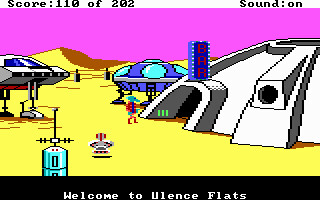The image is a screenshot from an old, colorful video game with a cartoon setting, portraying an alien landscape. At the top of the screen, a small white box displays a score of "110 out of 202" on the left and "sound on" on the right in black text. The bottom of the screen features a small black box with white lettering that reads, "Welcome to Eulens Flats." The game scene itself depicts a tan, dirt-covered ground with a lavender sky, hinting at an outer space environment. Prominently, a small alien creature stands in front of a grey dome-shaped building marked with a dark red "BAR" sign, which has a light blue and dark blue slogan. Nearby, a couple of robot-like creatures are seen on the ground along with two spaceships: one silver and square-fronted, the other circular and blue. The setting resembles a desert landscape on some distant planet or outpost.